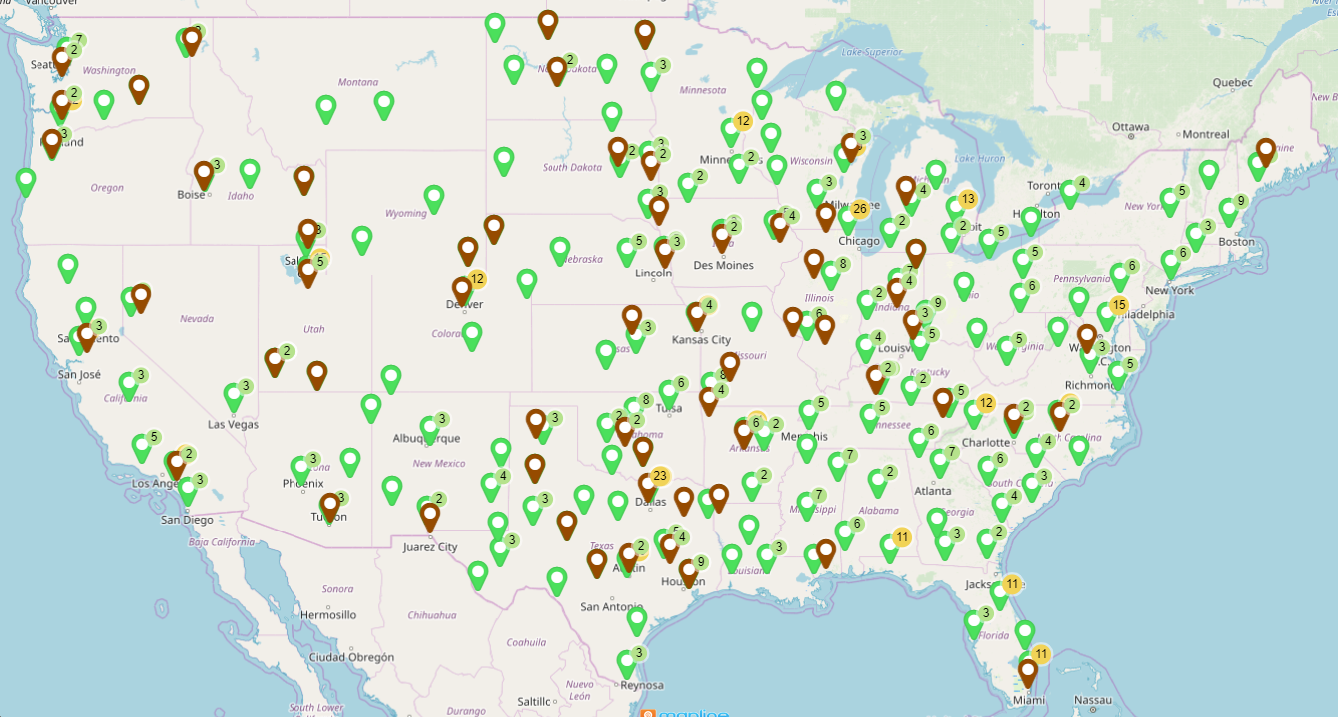This map of the United States displays states with distinct outlines and features various markers in different colors. The map itself has a grayish-pink hue. Scattered across it are place markers resembling those typically used to indicate locations on a map. These markers come in several types: green dots with white centers, brown dots with white centers, yellow circles with black numbers, and green circles with black numbers.

There is a higher concentration of these markers on the eastern side of the country compared to the western side. The green markers appear both along the east and west coasts, suggesting these might represent significant cities or perhaps important locations.

Specific cities identified with markers include:
- New York City
- Possibly Albany and Hartford-Springfield in Connecticut
- Boston
- Philadelphia and possibly Pittsburgh in Pennsylvania
- Richmond in Virginia
- Columbus in Ohio 
- In the west, markers in Montana likely denote Billings and Bozeman 
- In California, markers appear to highlight San Diego, Los Angeles, and San Francisco along the coast.

The precise meaning of these markers is unclear, although they seem to indicate major urban areas or possibly key locations within each state.